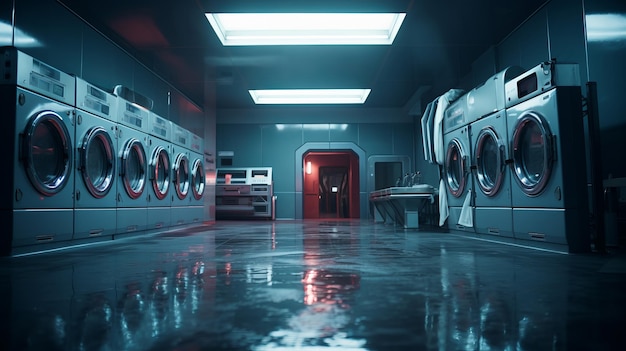This image, likely a screenshot from a movie or TV show, depicts the eerie setting of a laundromat taken from a ground-level perspective. Dominated by an unnatural blue hue, possibly from a filter or specific lighting, the scene exudes an unsettling atmosphere reminiscent of a horror film. The laundromat's floor, glossy and reflective as if wet, mirrors the six front-loading machines lined up on the left and the three on the right, each characterized by wide metallic doors with porthole windows framed in silver. The machines have a vertical orientation with distinct sections separated by black spaces. Above, fluorescent lights hang, casting a stark blue glow across the stark white and blue-tinted room. The background features additional metal shelving or possible seating, flanked by an arched doorway that leads into a series of rooms and hallways bathed in an ominous red light — the only warm color in an otherwise cold scene. The back wall of the laundromat is covered in large blue tiles, adding to the monochromatic and somber feel of the image.